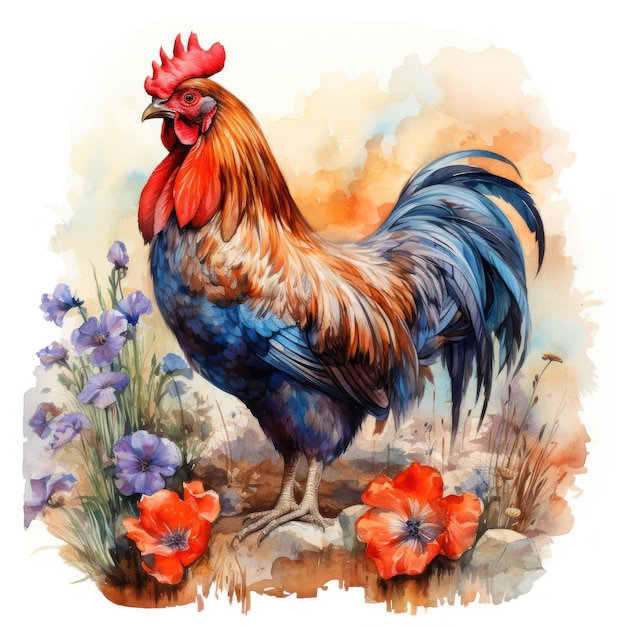This watercolor painting features a vibrant rooster facing left. The rooster's striking red comb with four spikes sits atop its brown head, accompanied by red feathers and a bright yellow beak. Red feathers also surround its eye. Its chest and lower feathers display a rich palette of dark blue, light blue, and occasional black. The back feathers are an array of white, bright yellow, and dark orange, contrasting beautifully with its light and dark blue tail feathers. The rooster stands on a small rock, its light gray legs and sharp nails visibly supporting it. Surrounding the rooster are two purple flowers positioned to its left and two orange flowers at its feet, with green stems and a touch of weeds interspersed. The background is a wash of light orange, reminiscent of colors bleeding on wet paper, while the rest of the backdrop remains white, emphasizing the rooster and the flowers.